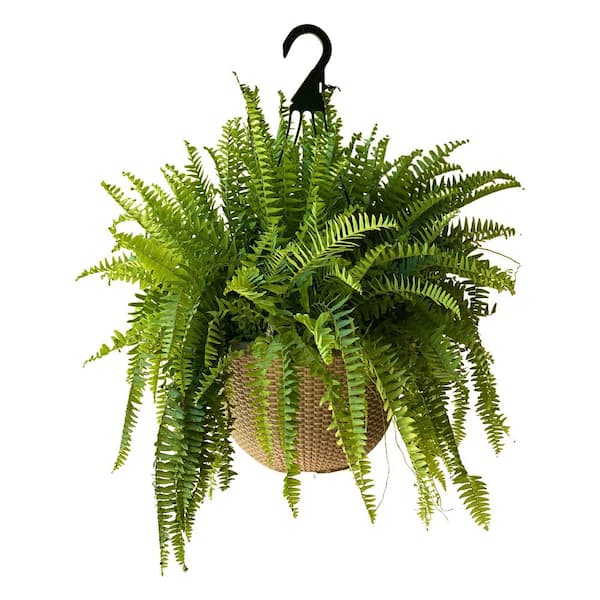A light beige ceramic pot is adorned with a lush arrangement of vibrant green ferns, each featuring a distinctly spiky exterior on their leaves. The ferns cascade gracefully over the edges of the pot, giving the plant a traditional and elegant appearance. Completing the aesthetic, a black handle is positioned at the top of the pot, adding a contrasting touch to the overall design.